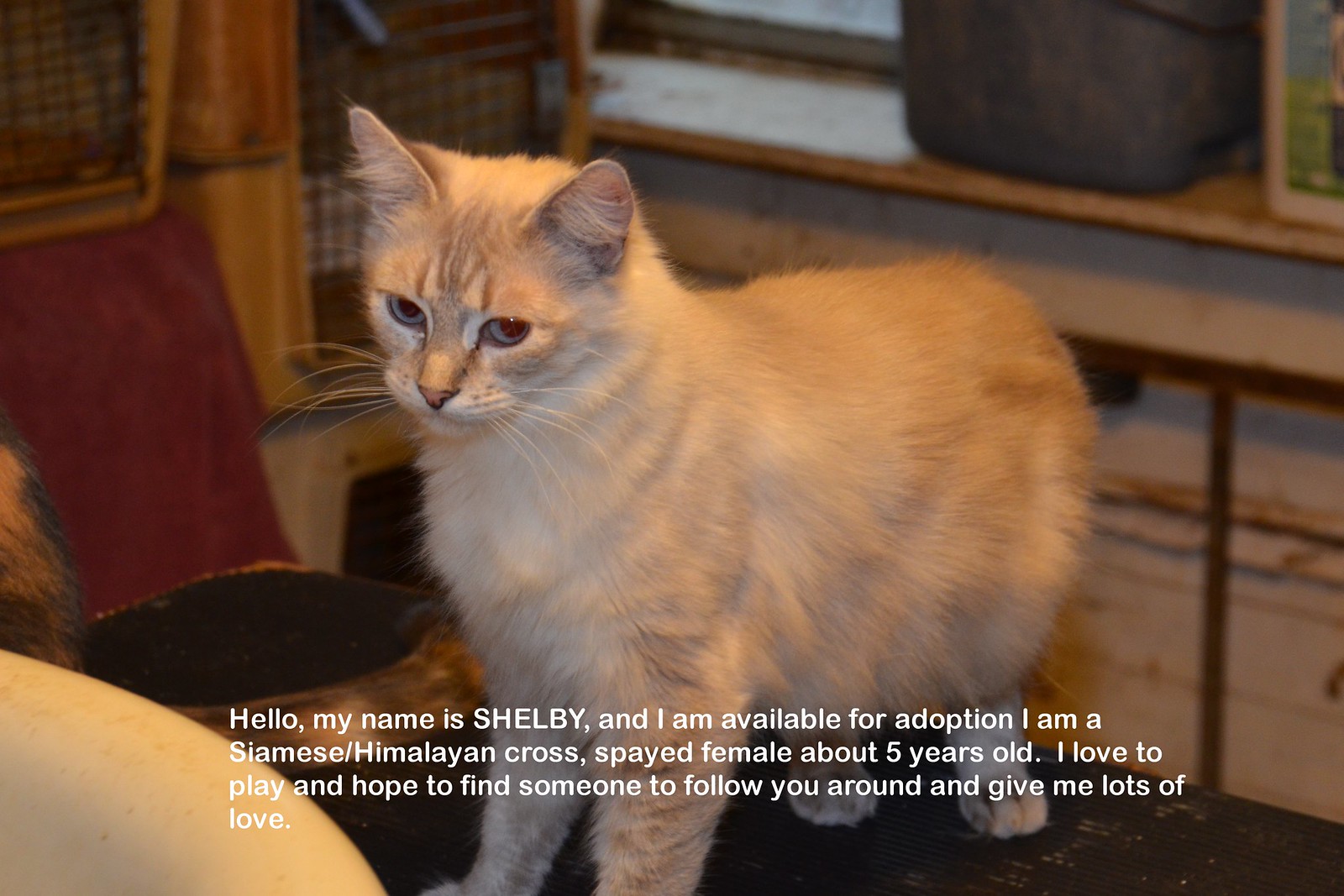In this indoor photograph, a cream-colored cat with blue eyes stands on all fours atop a small table. The cat, identified in the text as Shelby, is a 5-year-old Siamese and Himalayan cross-bred female available for adoption. The lighting suggests it's daytime, with a beam of light illuminating Shelby as she stands in the center of the image, slightly angled with her face to the left and her tail to the right. In the background, a chair is visible along with stacked crates or kennels on one side and a metal table with some buckets on the other. The setting includes various household items, adding to the homely atmosphere. At the bottom of the image, white text reads: "Hello, my name is Shelby and I am available for adoption. I am a Siamese/Himalayan cross-bred female, about 5 years old. I love to play and hope to find someone to follow you around and give me lots of love." This photograph appears to serve as an advertisement for pet adoption, highlighting Shelby's playful nature and readiness to find a loving home.